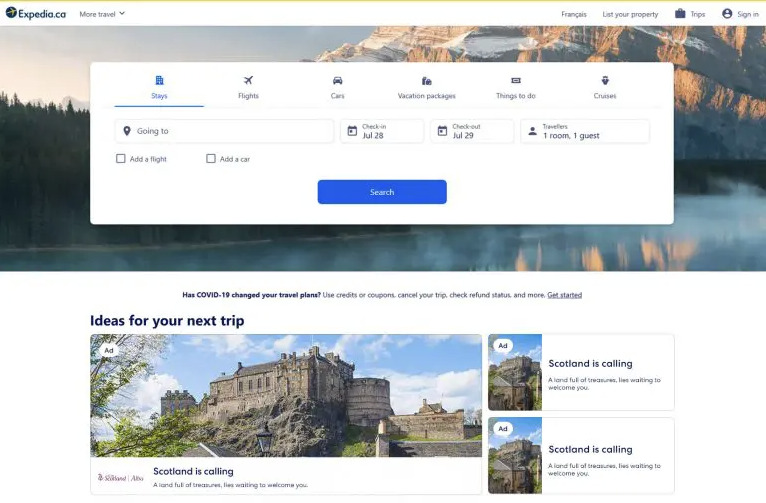The screenshot captures the Expedia.ca website, with its interface showcasing various travel options and features. In the top-left corner, the Expedia logo is prominently displayed. Adjacent to it on the right, there's a dropdown link labeled "More Travel." Further right, the website offers a language switch option indicating "Français," signifying a French language option. Next to it is a "List your property" link, followed by a "Trips" section accompanied by an icon resembling an attaché case. The row concludes with a "Sign In" option.

Beneath this top navigation bar, a stunning screensaver image of the Yosemite mountains is displayed, featuring a serene lake in the foreground. Centered below this image are several tabs for different types of travel services: "Stays" (currently selected), "Flights," "Cars," "Vacation Packages," "Things to Do," and "Cruises."

Directly underneath these tabs is an input field labeled "Going to," complete with a locator icon. Next to it, the check-in date is set to July 28th, marked by a calendar icon, and the check-out date is July 29th, indicating a one-night stay. Further to the right, the traveler information specifies "1 room, 1 guest."

Beneath these input fields are two square buttons, allowing users to add a flight or car to their booking. Dominating the center of the layout is a prominent blue "Search" button.

Towards the bottom of the screenshot, there's a message addressing COVID-19's impact on travel plans, offering options to use credits or coupons, cancel trips, check refund statuses, and more, with a "Get Started" hyperlink.

Finally, another grand image showcases a picturesque view of Scotland, accompanied by the text "Scotland is calling." Below this, a caption reads, "A land full of treasures, lives waiting to welcome you," inviting travelers to consider Scotland for their next adventure.